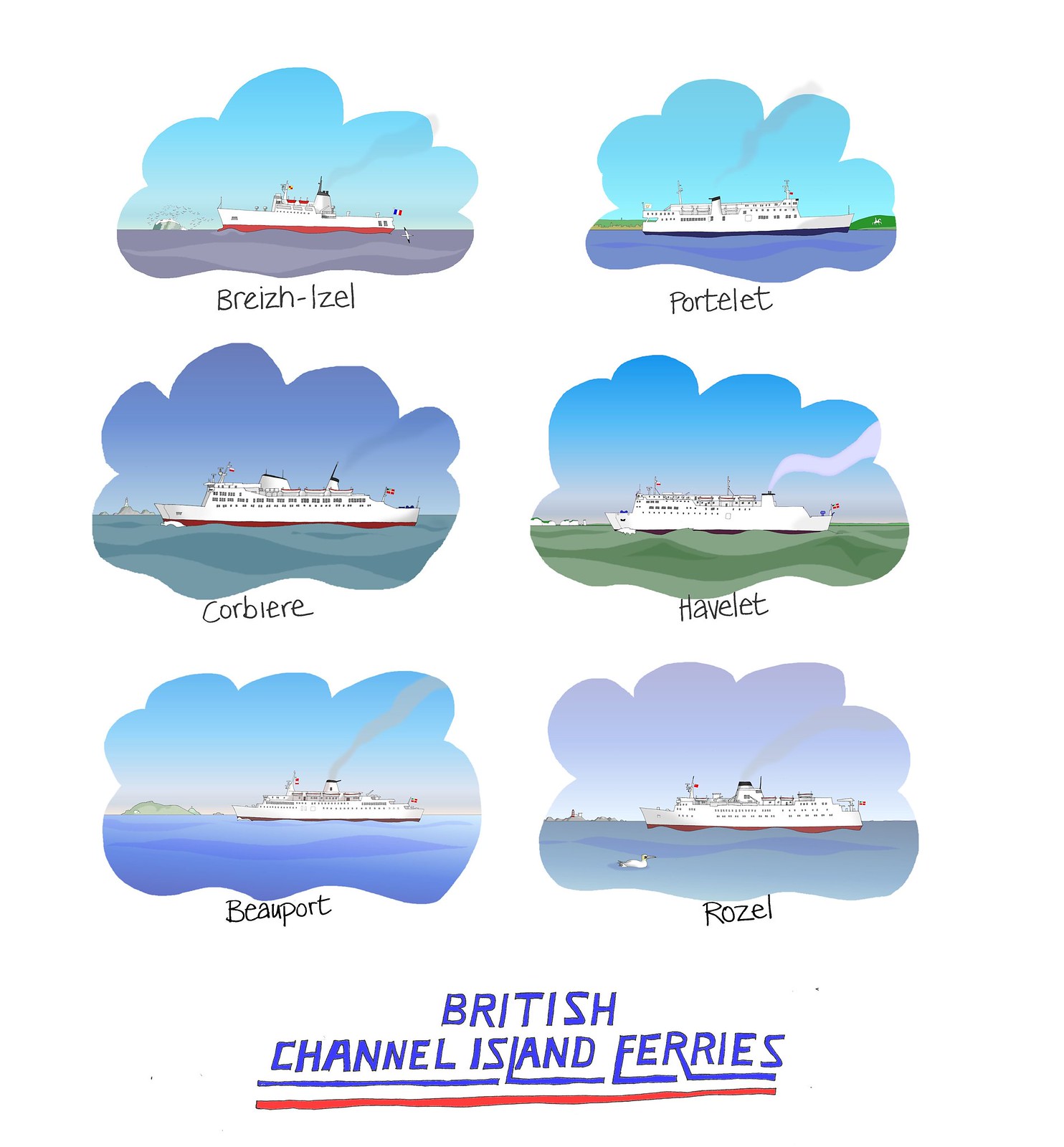The poster, serving as an advertisement for British Channel Island Ferries, features a white background adorned with six cloud-shaped illustrations, each enclosing a different ferry. These cloud shapes have scalloped edges and display a serene scene with a blue sky and ocean, stylized in a cartoonish manner. The ferries' names are written in black text beneath each corresponding illustration: Bryse Iselle, Portelet, Corbiere, Havalet, Beauport, and Roselle. Arranged in three rows and two columns, the vividly depicted ferries stand out with their varying details, including different colored hulls with some sporting red or black bottoms. At the bottom of the poster, the text "British Channel Island Ferries" is prominently displayed in bold, blue, block letters—each letter's base extended to form a blue underline further emphasized by a red line below it. This vibrant design aims to catch the viewer's eye and inform them about the diverse fleet of the British Channel Island ferries.